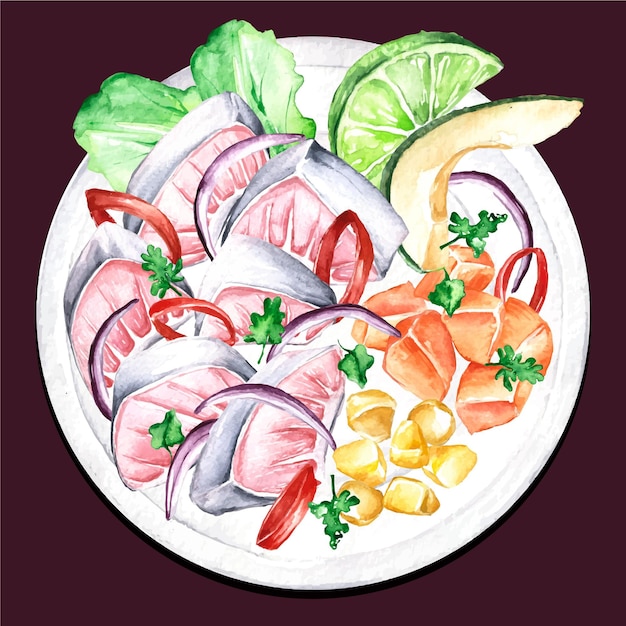This detailed hand-drawn image features a white plate positioned centrally and facing the viewer, brimming with an assortment of fruits and vegetables. The background is distinctly bifurcated, with the upper half in dark purple and the lower half in light purple. At the top of the plate, progressing from left to right, there are two green lettuce leaves followed by a half-sliced green lime. Nestled in front of the lime is a slice of cantaloupe, characterized by its tan interior and green outer layer. Beneath the lettuce, extending to the bottom of the plate, are several slices of watermelon with a striking red center surrounded by a thick blue rind. Scattered on and around the plate are four slices of purple-red onion and a handful of red pepper rings. Toward the bottom corners, clusters of six small yellow corn kernels can be found, accompanied by six orange-hued cubes, possibly a form of cut-up chicken or sweet potato. The plate is also adorned with sprigs of green herbs that add a fresh touch throughout.